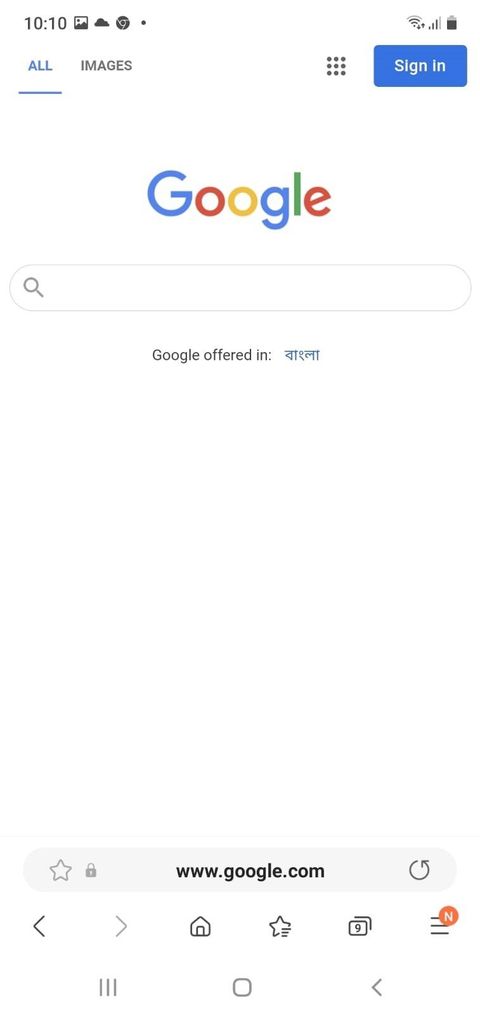A detailed screen capture from an iPhone displaying the Google search app interface. The standard iPhone status bar is present at the top, showing the time (10:10 AM), signal strength, and battery level icons. The bottom part of the screen features the typical iPhone navigation buttons, including "Close All," "Close," and "Back."

The Google app is open but no search terms have been entered. The familiar "Google" logo sits at the top of the screen, above a blank search field. Beneath the search field, there is a message that reads "Google offered in" followed by some Asian characters, suggesting language options. In the upper right corner next to the search bar, a blue "Sign In" button is visible. To the left, an “All” link is underlined in blue, indicating the current tab, with an "Images" tab adjacent to it.

Towards the bottom, the URL "www.google.com" is displayed prominently. The main portion of the screen, predominantly white, reflects the absence of search results or any entered search parameters. In the lower right corner, an indicator shows there are nine messages waiting to be reviewed. 

Overall, this screen capture depicts a clean and basic view of the Google app's homepage on an iPhone, before any search activity has taken place.